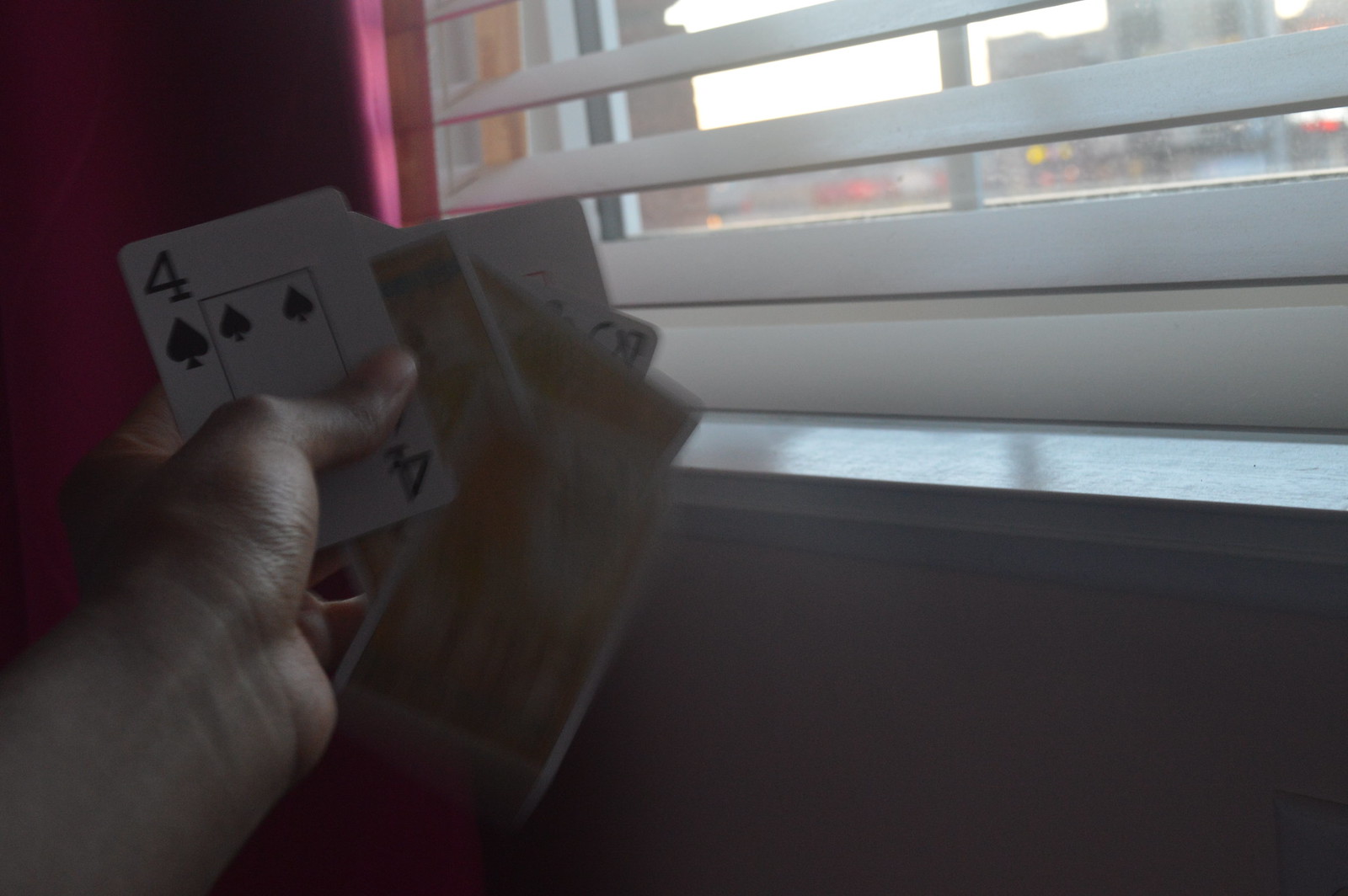A close-up, slightly blurry image captures a person holding a fan of playing cards in their left hand. The perspective suggests that the photo was taken from the viewpoint of the cardholder, possibly with their right hand. The thumb and most of the hand are visible in the bottom left corner, tightly gripping a set of cards. The card at the forefront is the four of clubs, distinctly marked with black symbols and numbers on a white background. The numbers "4" in black are located in the top left and bottom right corners, with the latter being upside down. The card displays three club symbols in black.

Behind the four of clubs are several more cards, arranged somewhat chaotically. The immediate next three cards show their backs, their faces hidden from view. Beneath these is a face-up card where only part of a three is visible, the rest obscured. The background features a pink wall and a window with partially open blinds, revealing a glimpse of sunny skies and distant buildings.